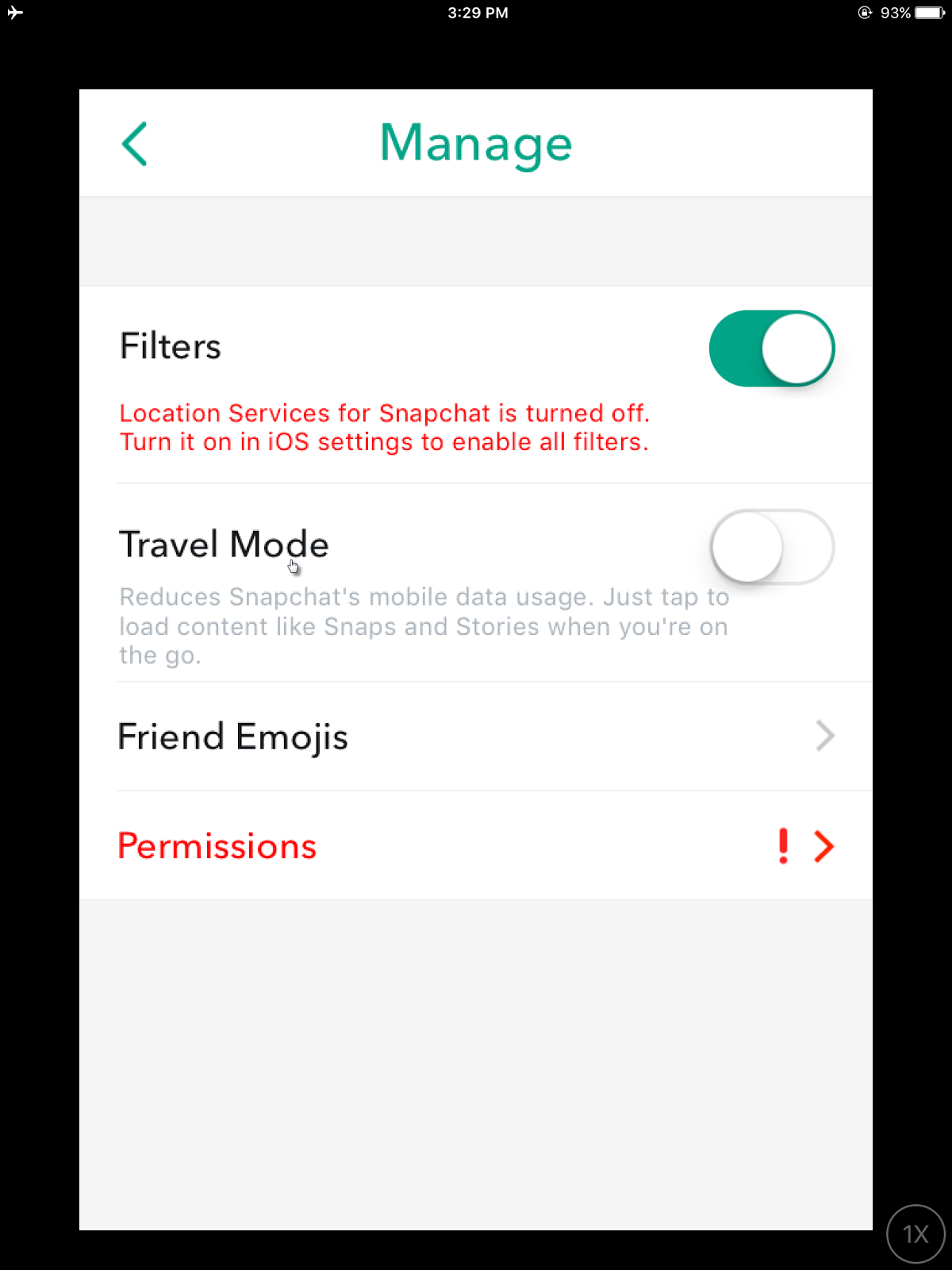This screenshot from a smartphone display showcases a typical interface with some unique elements. The background is a deep, pitch-black, devoid of any gray tones. At the very top, the time is displayed in a crisp white font as "3:29 PM." To the right of the time, the battery icon shows a 93% charge. On the opposite corner, a small airplane icon indicates that the device is in airplane mode.

Dominating the center of the screen is a pop-up box with a white background. At the top center of this box, the word "Manage" is displayed in an aquamarine green font, accompanied by an arrow on the left side. Below this header, there is a gray separator line.

Just underneath the gray line, the white background resumes, and it features the heading "Filters" in bold text. Following this, in red text, there is an alert that reads, "Location services for Snapchat is turned off. Turn it on in iOS settings to enable all filters." Adjacent to this message is a toggle switch, which has been slid to the right and turned aquamarine green, indicating that the setting has been activated.

Further down, the text "Travel Mode" is displayed in black. Beneath it, in gray text, a description explains, "Reduces Snapchat's mobile data use. Just tap to load content like snaps and stories when you're on the go." This particular setting shows as turned off, indicated by a white toggle.

At the bottom of the pop-up box, the text "Friend Emojis" appears in black, and below that, the word "Permissions" is prominently written in red. To the right of "Permissions," there is a red exclamation mark and a red arrow pointing to the right, signaling an important action item.